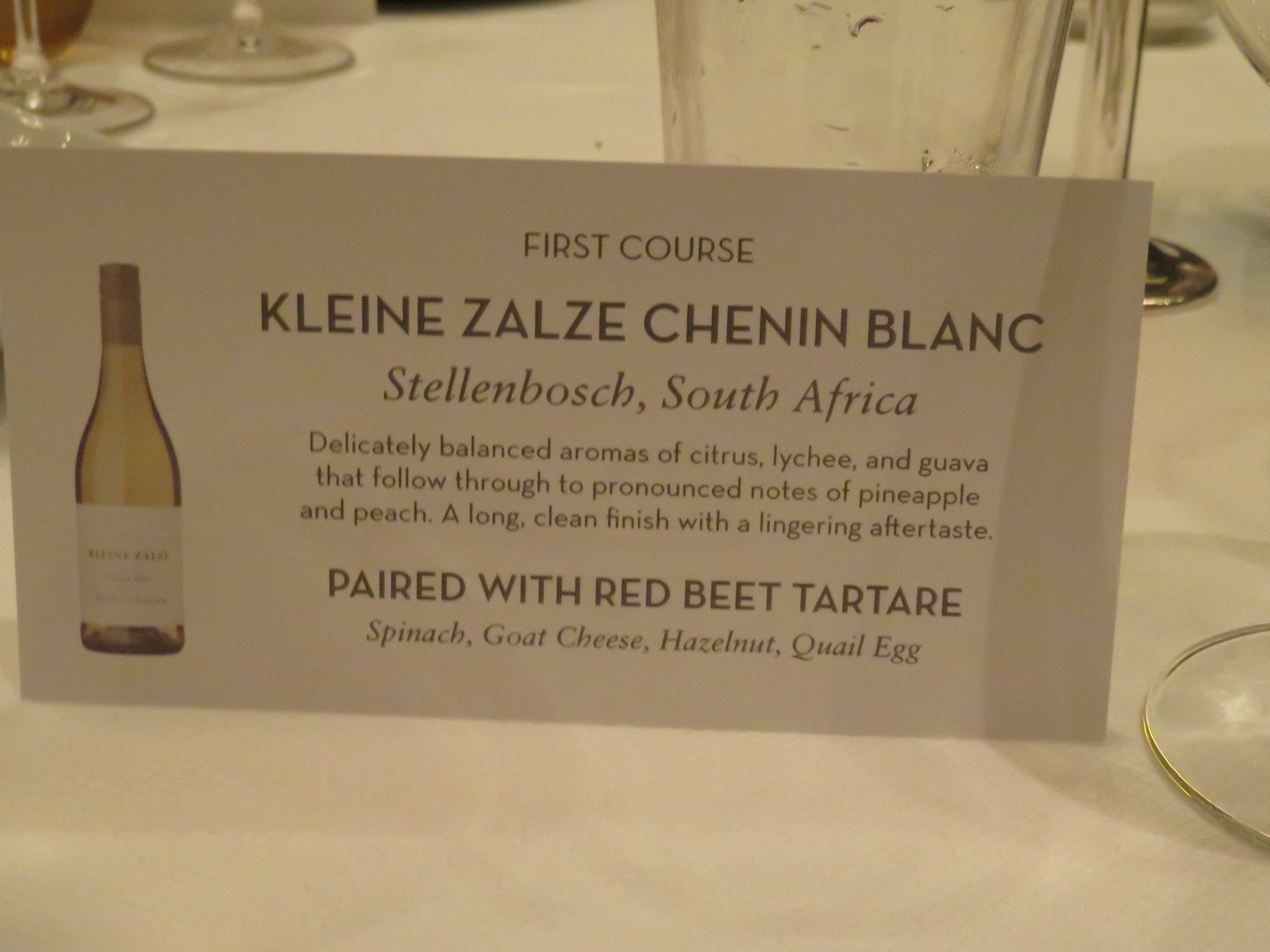The photograph is a close-up shot of a dining table set for a multi-course meal. Dominating the background are several stems of long-stemmed wine glasses, along with a pitcher. Leaning against the pitcher is a white card with blackish-brown print. The card features an image of a wine bottle on the left and details about the first course: "Kleine Zalze Chenin Blanc, Stellenbosch, South Africa." The description on the card highlights the wine's delicately balanced aromas of citrus, lychee, and guava, with pronounced notes of pineapple and peach. It promises a long, clean finish with a lingering aftertaste. The card also notes that the wine is paired with a dish consisting of red beet tartare, spinach, goat cheese, hazelnut, and quail egg.